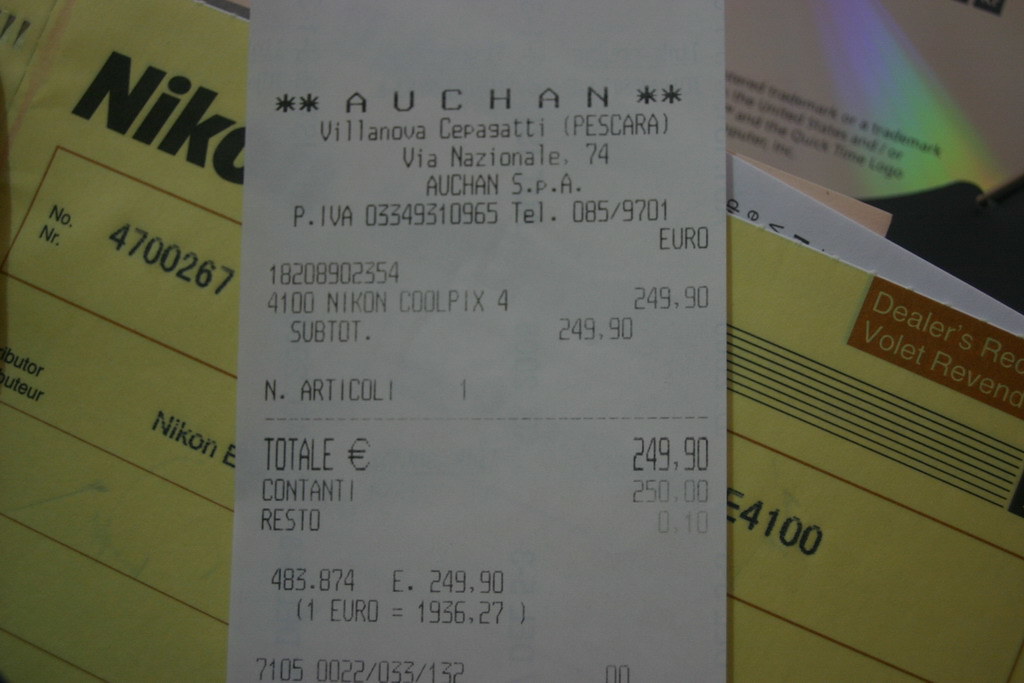The image displays an assortment of stacked papers, primarily a white receipt prominently positioned on top of a yellow warranty card. This white receipt, written in a foreign language, originates from AUCHAN and lists details such as the store address, phone number, and prices in Euros. It indicates a purchase of a Nikon Coolpix 4 for €249.90, with an additional note about a partial payment of €50 and a €0.10 charge-back. The receipt contains details like the item number 4100 for the camera. The yellow warranty card below also references the Nikon Coolpix, featuring the number 4700267, possibly a serial or transaction number. This yellow document is part of the warranty and manuals, which are arranged in a tilted orientation across other partially visible brown and white papers, creating a layered visual effect in the photo.